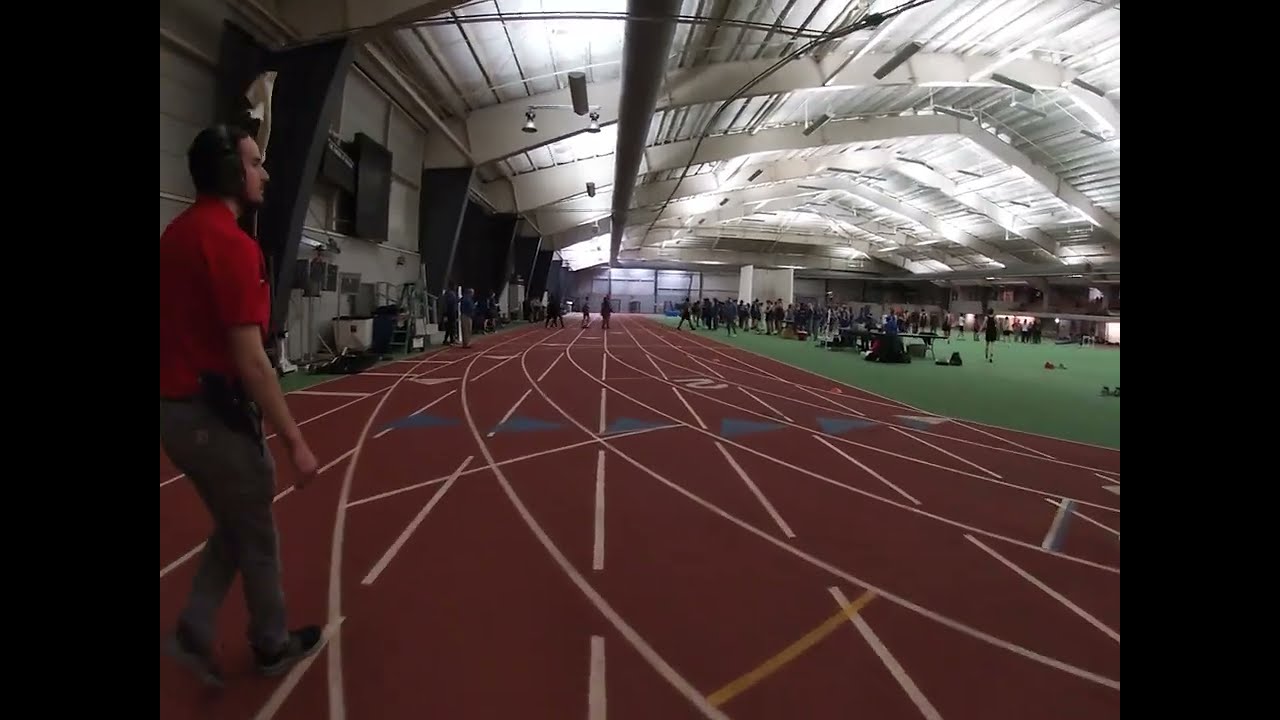The image depicts an indoor running track made of a tan synthetic material with white lines delineating each lane, along with numbers, white arrows, and blue arrows. The track surrounds a central green artificial turf field, where multiple people dressed in sportswear are gathered, possibly preparing for a race. The ceiling, composed of a thin white material and supported by white columns and beams, is illuminated by various fluorescent lights. On the left side of the image stands a man wearing a black headset, a red polo shirt, gray pants, and black shoes. A radio is clipped to the right side of his hip, suggesting he might be a race official or coordinator. The photo includes black bars on the left and right sides, giving it a letterboxed appearance. In the background, a few individuals can be seen standing on the track.